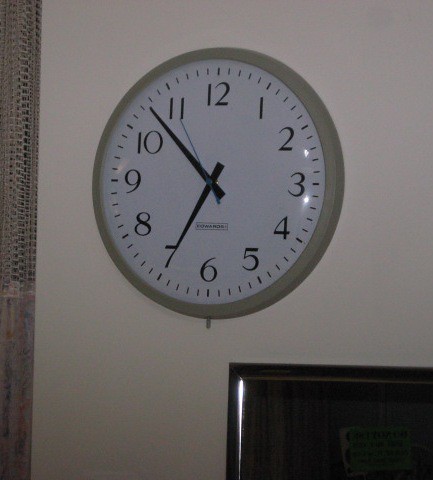The image depicts a generic clock hanging on a wall. The clock features a dark white frame and a white face with black numerals. It is equipped with a black hour hand, a black minute hand, and a striking blue second hand. On the bottom right side of the image, part of a closed, wooden doorway is visible. A piece of paper is posted at the center of this door. The corner where the door is located is somewhat darker. To the left side of the image, a shade extends from top to bottom, becoming semi-transparent near the top and more opaque, almost fabric-like, towards the bottom.